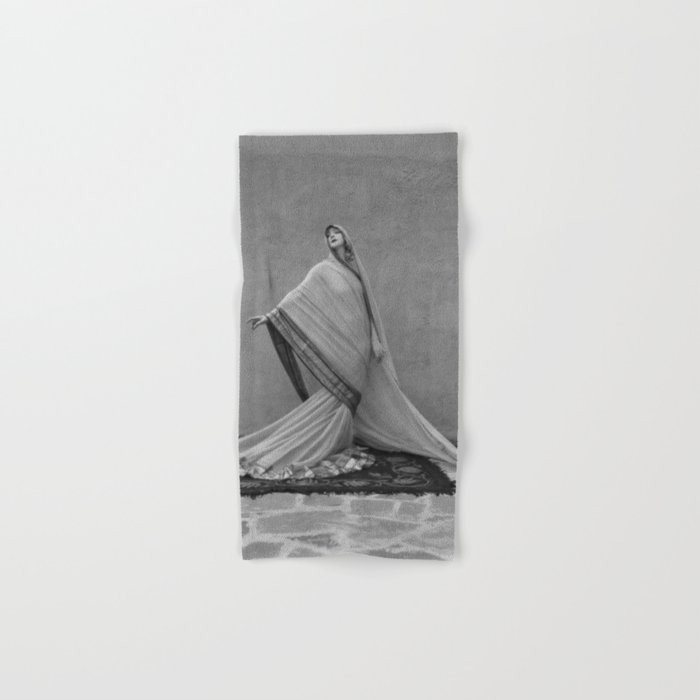This is a monochromatic illustration with a soft, light gray background. Dominating the vertical, rectangular image is a detailed, realistic drawing of a woman standing on an ornate rug, itself set upon a cobblestone street. She is dressed in elaborate ethnic attire, wearing a long, flowing dress and a shawl that drapes over her head and cascades around her body, evoking a sense of elegance and modesty. The woman is depicted standing in front of a darker gray wall, her arm gracefully outstretched and pointing to the left, as she gazes in that direction. The intricate textures and patterns of the rug, as well as the meticulous detailing of the woman’s clothing, suggest that the illustration may have been created using graphite or charcoal, capturing a serene and timeless moment.